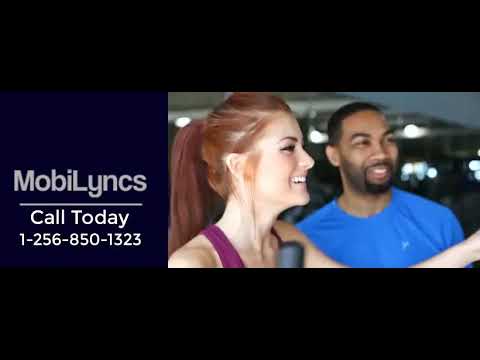In this promotional image for MobiLynx, on a predominantly black background, the right side features a vibrant photograph of a woman and a man seemingly enjoying their time at night. The woman, a white female with red hair tied in a single ponytail, is dressed in a sleeveless purple tank top. She is smiling broadly, showing her top row of teeth, and is looking to the right with her left hand raised and bent in the same direction. Next to her, the man, who appears to be either Black or Hispanic, sports a closely trimmed beard and mustache forming a square shape outline. Dressed in a blue shirt, he is also smiling and looking in the same direction as the woman. Both appear to be posing professionally, complete with makeup, against a backdrop that hints at lights in the distance, adding to the lively ambiance. The photo suggests they might be at a gym, as indicated by what seems to be the handle of an elliptical machine in the foreground. 

On the left side of the image, gray text on a black background prominently displays "MobiLynx" with the letters 'M' and 'L-Y-N-C-S' capitalized. Below this, white text instructs viewers to "call today," followed by the phone number 1-256-850-1323. The clear and professional arrangement of the photo and text makes it evident that this image is part of an advertisement campaign for MobiLynx.